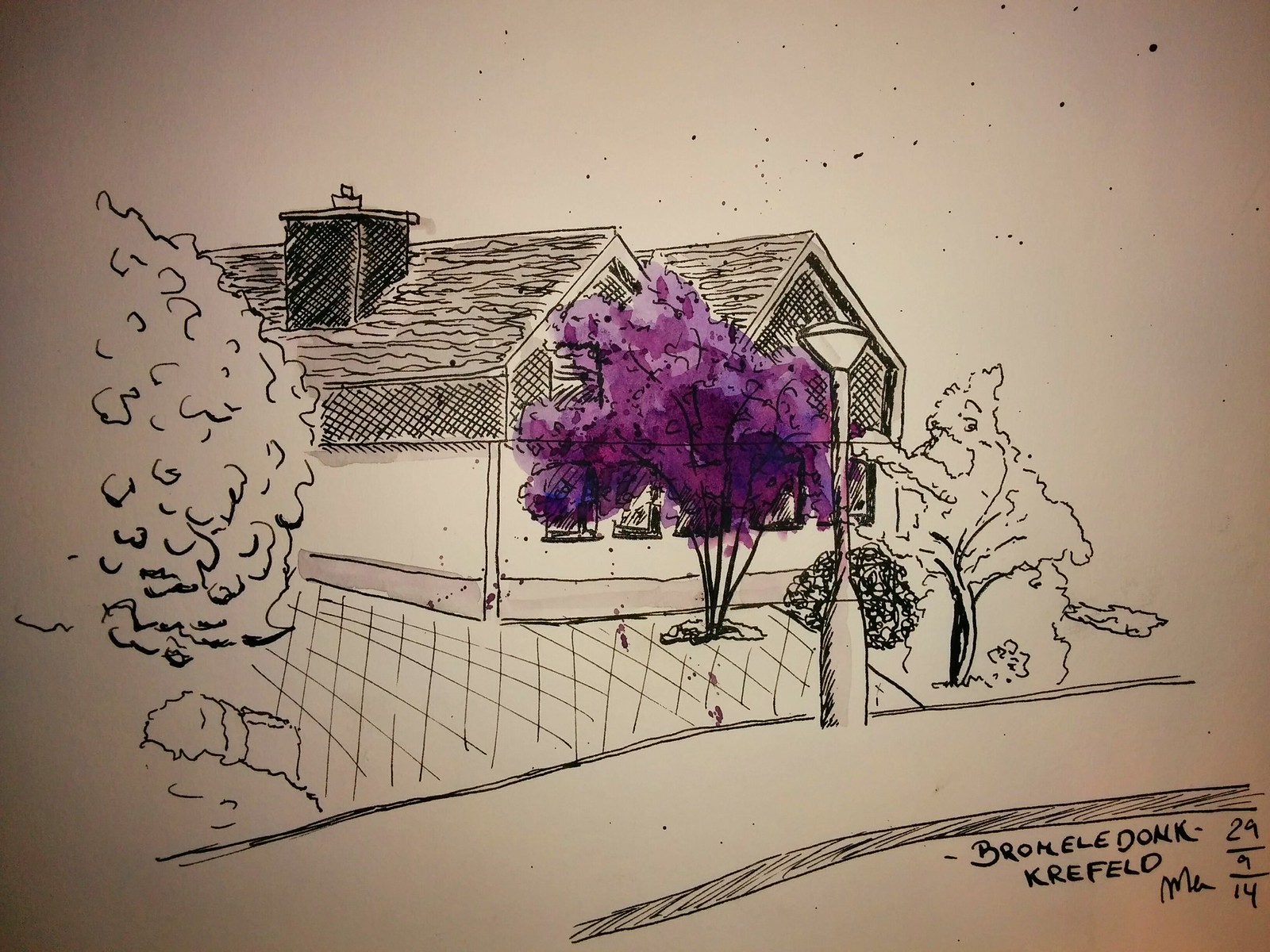The image depicts a detailed black-and-white sketch on a white piece of paper. The central focus is a two-story house with two peaked roofs, complemented by multiple trees and shrubs surrounding it. The intricate shading of the roof showcases subtle brown hues and horizontal lines, with a small, slightly elevated chimney marked in dark shades with white specks. The upper part of the house is crosshatched, giving it a textured appearance, while the lower walls remain predominantly white with gray trim at the bottom. 

In front of the house, there is a unique purple tree, the only element in color, providing a striking contrast against the monochromatic backdrop. The tree features a black base with its leaves and branches in a rich purple gradient, dominating the foreground and partially overlapping the house. A street lamp, roughly one story tall with a V-shaped light and dome top, stands just right of center, adding to the foreground elements. To the left, crisscross and squiggly lines represent a lawn and a tall bush or tree, respectively.

Additionally, a sidewalk traverses the left side of the drawing, extending into the scene but not reaching the image's edge. The presence of other, smaller bushes and trees, all rendered in black, enhances the scene's depth and composition. At the lower right corner, the inscription "Bromley, Donk, Creffield" appears along with the date "29/9/14," likely indicating the artist's details and the date of creation.